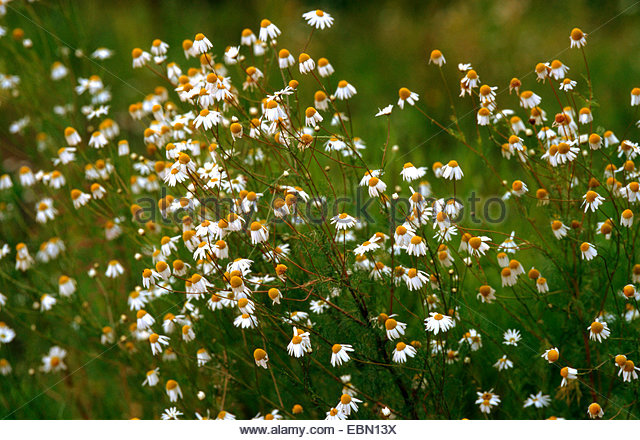The image depicts a close-up view of a field filled with small white-petaled flowers, possibly daisies, characterized by their downward-pointing petals and vibrant orange centers. The flowers are scattered across the left, middle, and right sides of the frame, with a denser cluster towards the left center. The background consists of blurred tall green grass, with hints of trees, adding a natural, verdant backdrop to the scene. Overlaid faintly in gray are the words "Alamy stock photo," indicating its stock image nature. At the bottom of the image, the text "www.alamy.com-ebn13x" is visible in black.